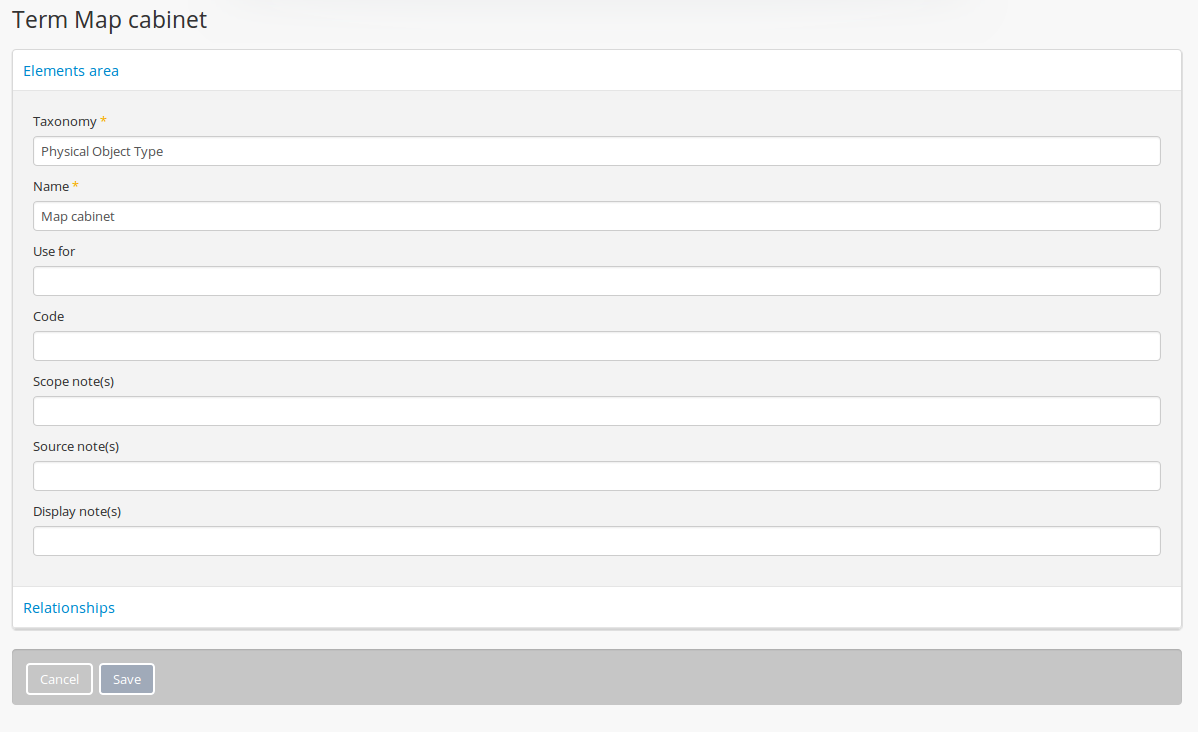The webpage features a nearly square, rectangular box with a very pale purple background. In a vertical arrangement, several white input fields are present for the user to enter various information.

At the top left, dark gray text displays the words "Term Map Cabinet." Directly beneath this, a long white box extends the width of the page; inside this box, the text "Elements Area" is prominently displayed in bright turquoise blue.

Below this header, the pale purple background shows the word "Taxonomy" with a gold asterisk to its right. The corresponding input box beneath contains the gray text "Physical Object Type."

Following this, the next input box is labeled "Map Cabinet," preceded by the word "Name" above it on the purple background, also featuring a gold asterisk.

The sequential entries continue with white boxes labeled "Use For," "Code," "Scope Notes," "Source Notes," and lastly, "Display Notes."

At the very bottom, a white banner spans the entire width of the screen, carrying the word "Relationships" in bright turquoise blue. Underneath, a dark gray banner runs across the page, featuring two buttons aligned to the far left. The "Cancel" button is defined by a white border and white text, while the "Save" button is a very dark gray, also with a white border and white text.